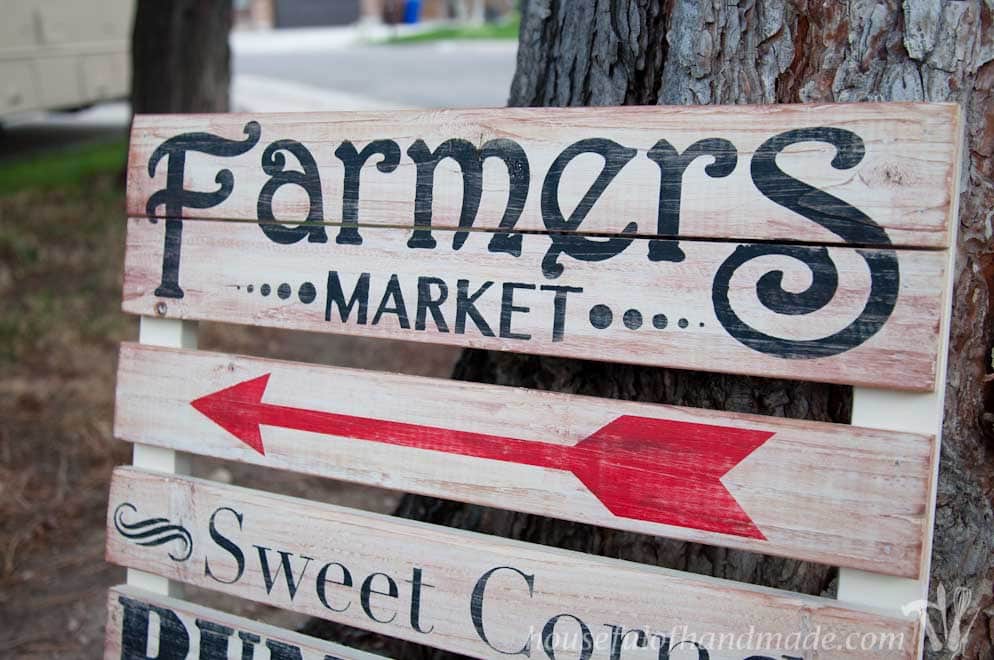A close-up image showcases a rustic wooden sign made from a whitewashed pallet resting against the trunk of a tree. The sign, painted in black lettering, reads "Farmer's Market" at the top across several slats, with "Farmer's" in a fancy script and "MARKET" in all capital letters below it, accompanied by decorative dots on either side. Below "MARKET," a red arrow points left. The next slat reads "SWEET CORN," but only the top of a few letters of the final word are discernible. The background includes a patch of grass, another tree to the left, and some pavement visible in the center. The image is taken outdoors during the daytime, providing a clear and brightly lit setting.